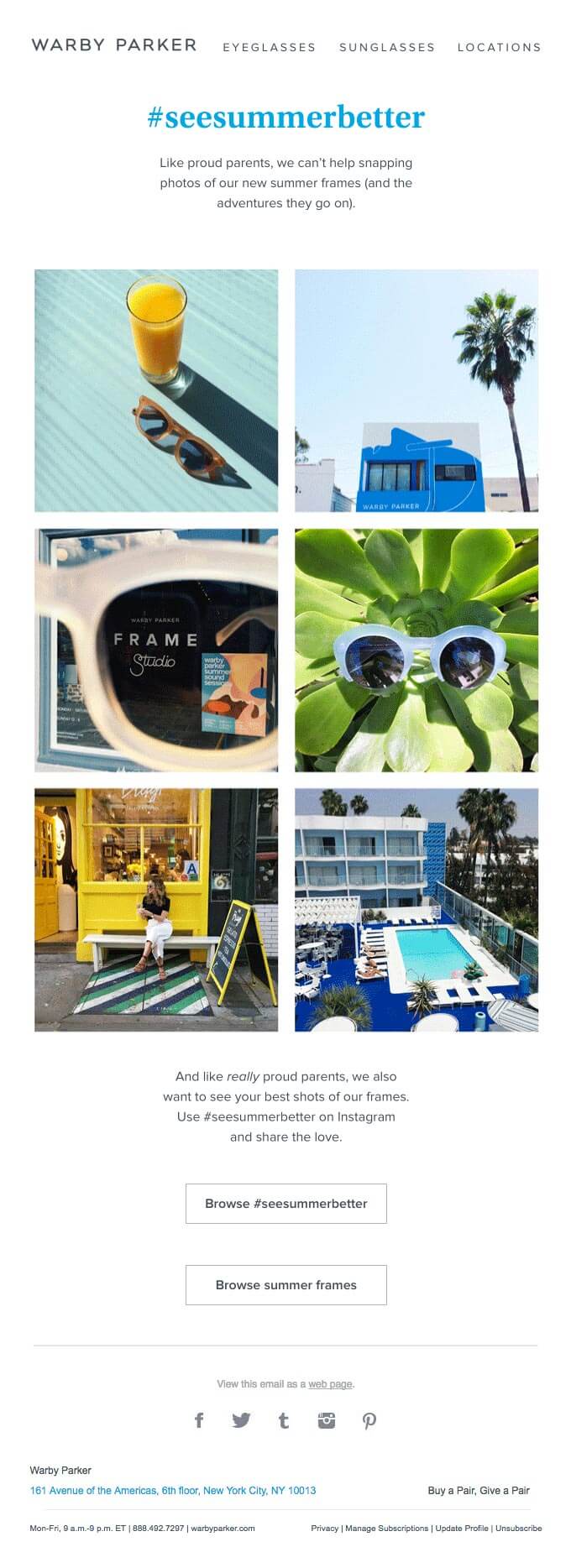Caption: 

"The homepage of the Warby Parker website is designed with a crisp, clean aesthetic. In the top left-hand corner, the name 'Warby Parker' stands out in a sleek dark gray or black font. To the right, visitors can easily navigate through three categories labeled 'Eyeglasses,' 'Sunglasses,' and 'Locations,' all displayed in the same dark font. The entire page is set against a pristine white background.

Beneath these categories, a light blue hashtag '#SeeSummerBetter' grabs attention, followed by a playful and proud message: 'Like proud parents, we can’t help snapping photos of our new summer frames (and the adventures they go on).' 

The layout then showcases six vibrant photos that embody the essence of summer, featuring Warby Parker stores, stylish sunglasses, and even a rooftop pool at a hotel. Each image complements the summery theme perfectly, creating a cohesive visual story.

Further down, another engaging blurb reads, 'And like really proud parents, we also want to see your best shots of our frames. Use hashtag #SeeSummerBetter on Instagram and share the love.' 

Finally, two inviting buttons at the bottom encourage visitors to 'Browse #SeeSummerBetter' and 'Browse Summer Frames,' making it easy to explore the latest seasonal offerings."